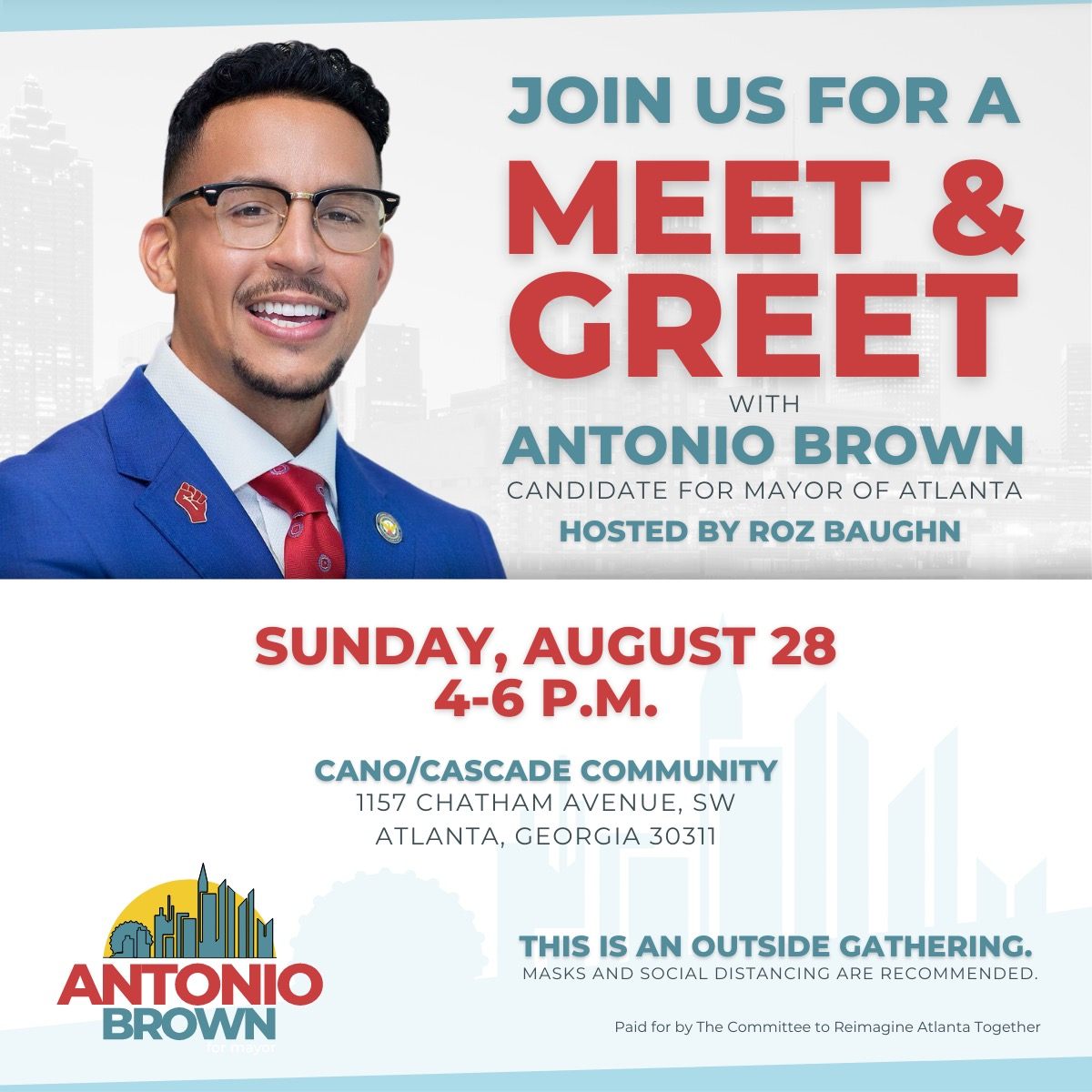The image is a detailed promotional poster for a political event featuring Antonio Brown, a candidate for Mayor of Atlanta. On the left side of the poster is a smiling Antonio Brown, dressed in a royal blue suit jacket, a red tie, and a white collared shirt. He has short black hair, glasses, a dark mustache, and a goatee. He is also wearing two lapel pins; one depicting the state of Georgia and another that is round but not clearly decipherable.

On the right side of the poster, bold text invites attendees to "Join us for a meet and greet with Antonio Brown," with "meet and greet" highlighted in red, and "with Antonio Brown" in blue or green. The text below states he is a "Candidate for Mayor of Atlanta," and the event is hosted by Roz Bond. Further details indicate the event will take place on Sunday, August 28th from 4 to 6 p.m. at Canoe/Cascade Community, located at 1157 Chatham Avenue, Southwest Atlanta, Georgia. An additional note specifies that the gathering will be held outdoors, with masks and social distancing recommended, suggesting the event might have been organized during the COVID-19 pandemic. The lower-left corner of the poster features a logo with Antonio Brown's name and a graphic of a city skyline within a yellow circle.